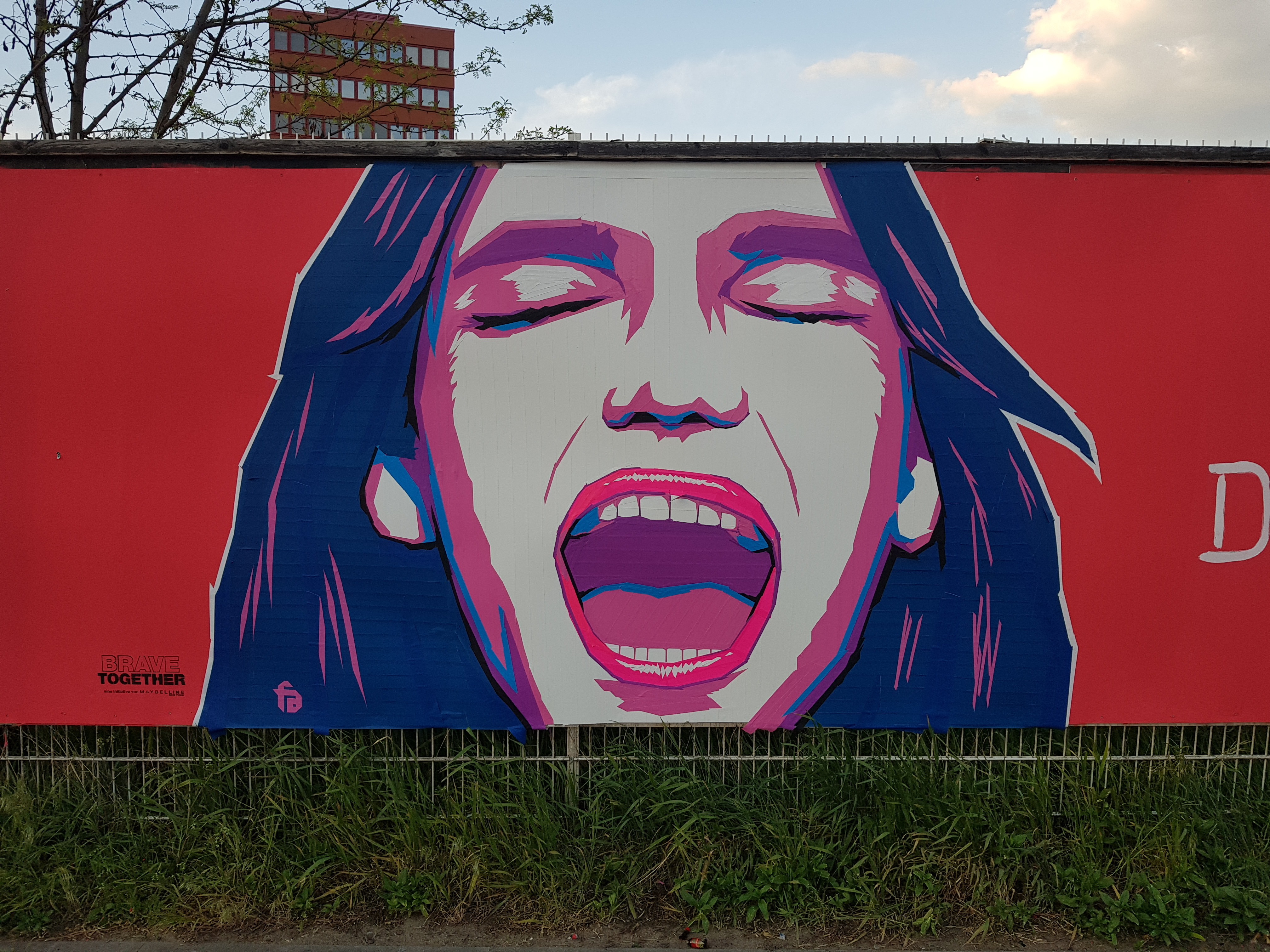The photograph captures a vibrant outdoor mural on a wall with a bright red background. The centerpiece of the mural is an abstract, vector-style illustration of a woman's head, rendered in shades of white, purple, blue, fuchsia, and pink. The woman, with long dark brown hair, has her eyes closed and her mouth wide open, revealing her red lips, teeth, and tongue, creating an impression of her either screaming or singing. This artwork, imbued with strong emotion, is not highly realistic but has a cartoonish and expressive quality.

To the left of her head, the mural features the text "BRAVE TOGETHER" and a white letter "D" on the right-hand side, though the photo is cropped so we only see a portion of this letter. The mural itself is large, giving the impression of a significant piece of street art, likely created with acrylic paint. Below the mural, a patch of overgrown green grass adds a natural element to the scene.

In the background, the sky is visible with white clouds, and the upper three floors of a brown building can be seen, partially obscured by a tree, which brings a sense of depth and context to the image.